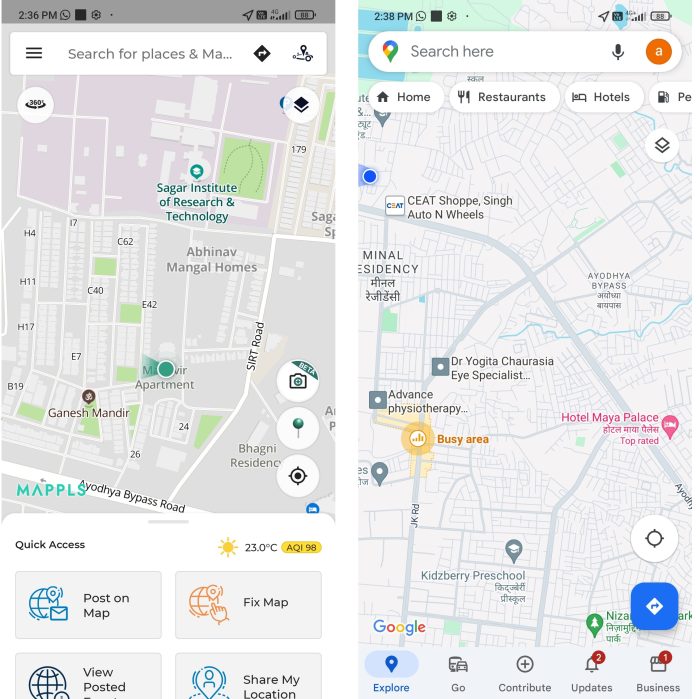This image showcases a side-by-side comparison of two mobile mapping applications, Map LS and Google Maps.

On the left side, the Map LS app interface is displayed. It features a search bar at the top of the screen for user queries. The label "Map LS" is positioned in the bottom left corner. Below the map area, there is a section labeled "Quick Access," which includes four distinct boxes: "Post on Map" and "Fixed Map" in the top row, and "View Posted" and "Share My Location" in the bottom row.

On the right side of the image, a screenshot of Google Maps is provided, which appears to be from a different location. "Google" is marked at the bottom left corner, and a blue navigation button with an arrow is visible at the bottom right. The bottom header menu includes five icons: "Explore," "Go," "Contribute," "Updates," and "Business." The "Updates" and "Business" icons have red notifications with numbers 2 and 1, respectively. At the top, there's a search bar that also features a microphone icon and a user profile image in a red circle. Below the search bar are three visible tags: "Home," "Restaurant," and "Hotel."